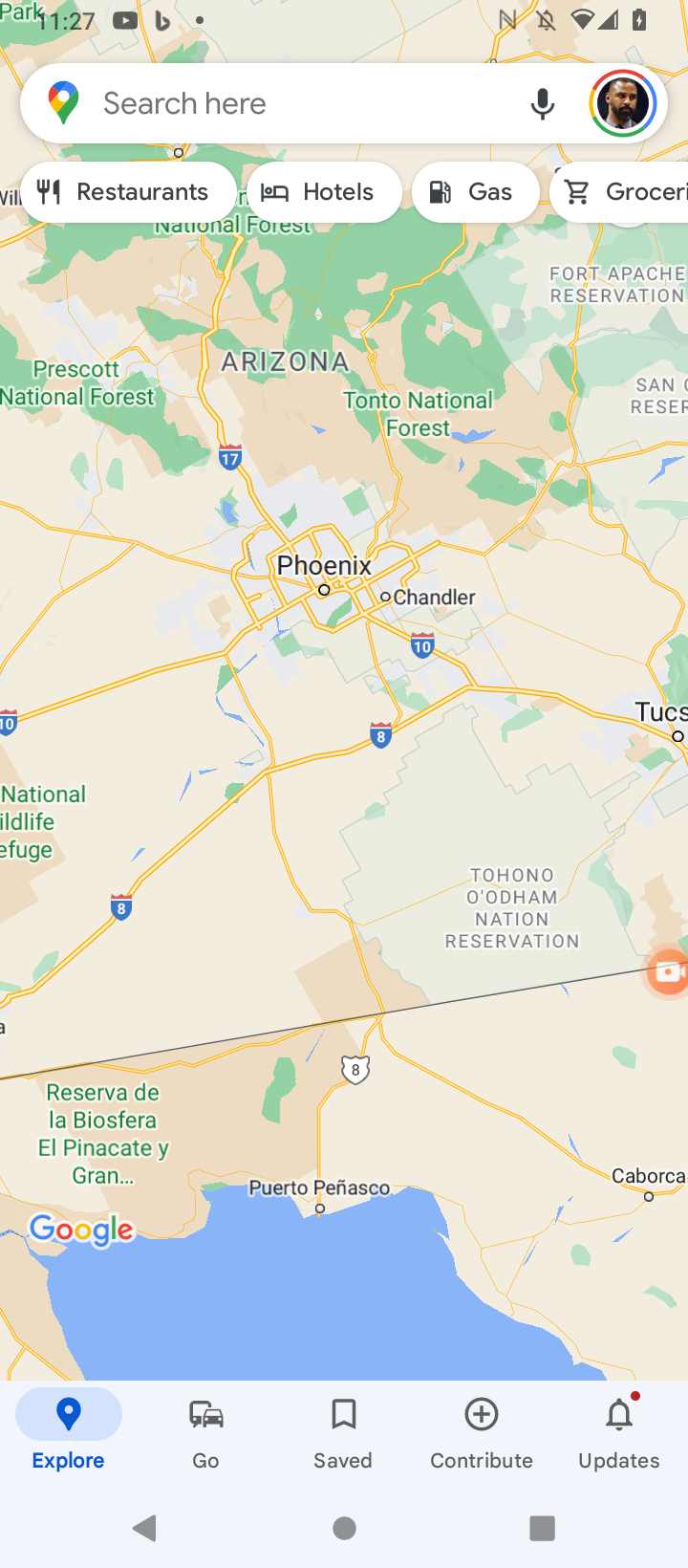A clear and descriptive caption for the image could be:

"This snapshot, taken from a cellphone, portrays a detailed map of Phoenix, Arizona, captured from Google Maps. At the top of the image, the phone's status bar is visible, showing the time as 11:27 and icons indicating folder, B, N, a crossed-out sound icon, internet connection, data connection, and battery status. The map prominently displays Phoenix and includes several other cities such as Chandler, Tucson, and Puerto Peñasco. Various geographical and administrative landmarks are also noted, including the Tonto and Prescott National Forests, as well as Highway 8 and Highway 10. The map extends southward to include parts of Mexico, featuring the Reserva de la Biosfera El Pinacate y Gran Desierto de Altar, and an Indian reservation, the Tohono O'odham Nation Reservation. Some parts of the map are difficult to read due to the small text size and partial cutoff."